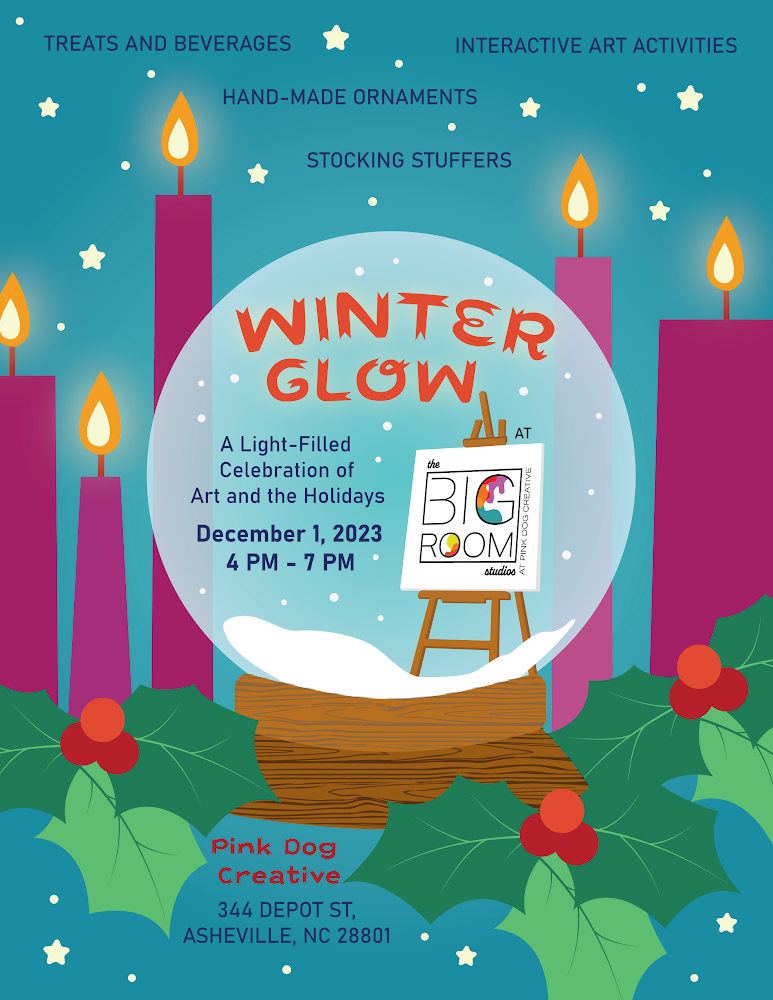This poster design advertises a public event set against a dark teal background sprinkled with light yellow stars that resemble snowflakes. The center showcases a computer-generated snow globe, semi-transparent with an orange handwritten font reading "Winter Glow." Inside the globe, in a smaller dark blue typewritten font, it states, "A light-filled celebration of art and the holidays, December 1, 2023, 4 p.m. to 7 p.m." Surrounding the snow globe, there are mauve-colored candles with cartoonish yellow and white flames emanating a subtle glow. Around the base of the globe and candles, holly leaves and berries add a festive touch. To the right of the globe, a wooden easel features a canvas inscribed with "Big Room Studios." Across the top of the poster, blue text lists event highlights: "Treats and beverages, interactive art activities, handmade ornaments, stocking stuffers." At the bottom, red text reads "Pink Dog Creative," with dark blue type underneath providing the address: "344 Depot Street, Asheville, North Carolina, 28801."